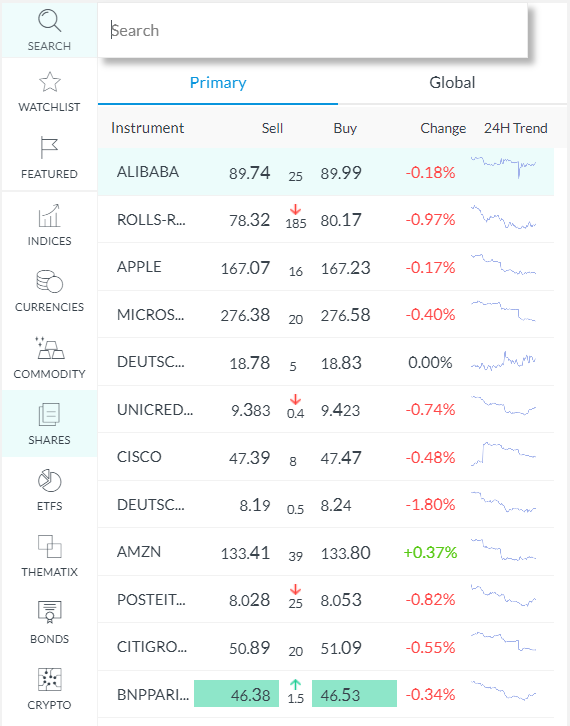The image is a screenshot from a mobile device displaying a financial market analysis app. The top left corner features a light blue "Search" label next to a white search bar. Along the left side, there are various sections accessible within the app including Watch List, Featured, Indices, Currencies, Commodity, Shares, ETFs, Thematics, Bonds, and Crypto. Among these sections, "Shares" is highlighted in blue, indicating it is the current selection.

At the very top of the screen, two tabs labeled "Primary" and "Global" are visible, with "Primary" being selected and marked by an underline in blue. The main display area is divided into columns titled Instrument, Sell, Buy, Change, and 24-Hour Trend. The box at the top lists "Alibaba" with a selling price of 89.74 and a buying price of 89.99. This entry shows a price change of -18%, displayed in red, and the entire Alibaba row is highlighted in light blue.

Towards the bottom of the screen, there's an entry for "BNP PARIBAS," presenting a selling price of 46.38 and a buying price of 46.53. These numbers are highlighted in teal green, drawing attention to them.